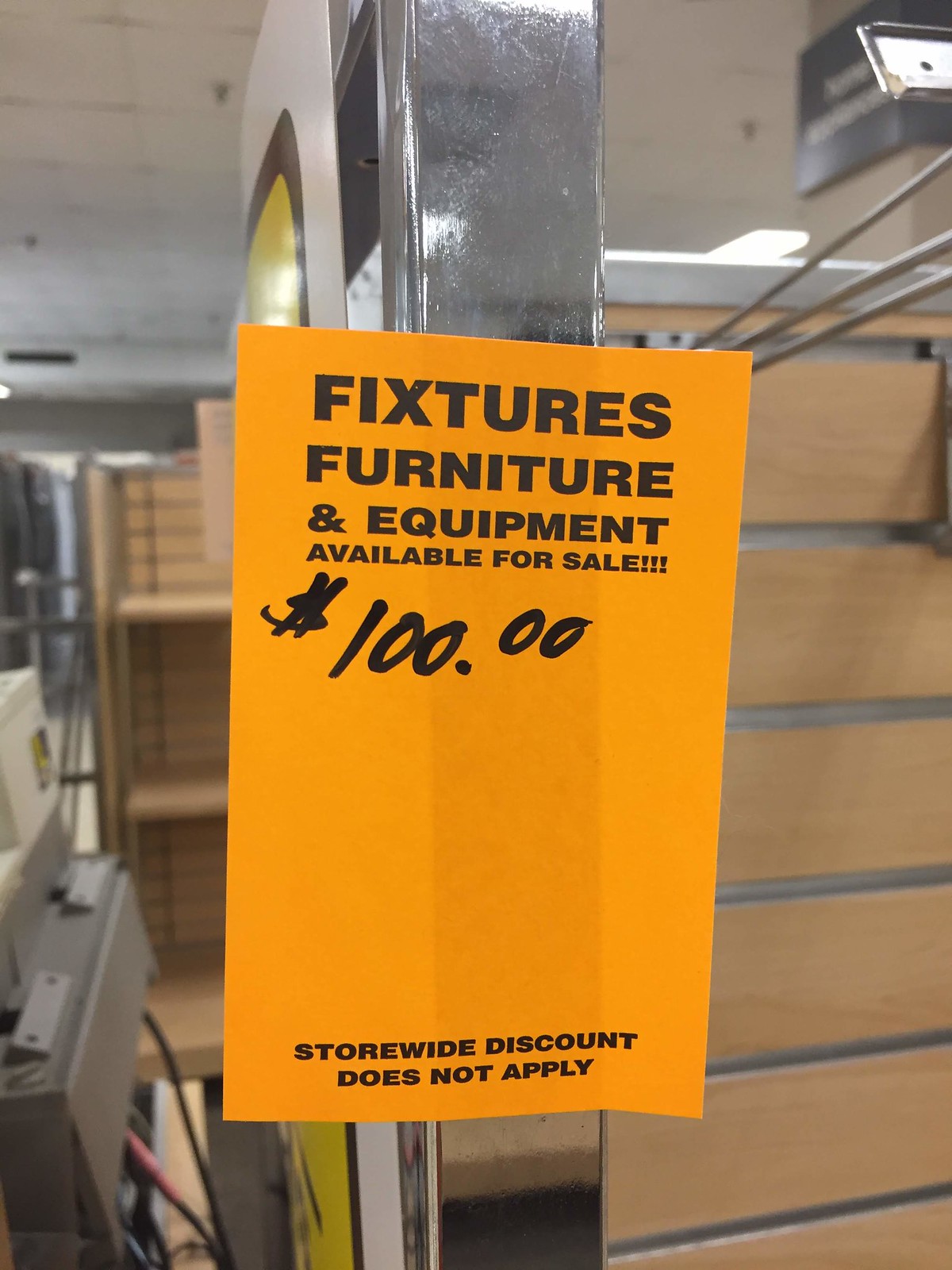This photograph captures a close-up of a neon orange sign in a store that's closing down. The sign, taped onto a silvery metal fixture inside the store, has bold black lettering that reads "Fixtures, furniture and equipment available for sale!!!", emphasizing the urgency and excitement of the sale. Below this, a handwritten note in black magic marker indicates a price of "$100." At the bottom, it states "store-wide discount does not apply" in black letters. The background reveals empty racks and shelves, suggesting the store’s inventory has been largely depleted. On the left side of the image, you can see what appears to be electrical or computer equipment, possibly a cash register, confirming the store's end-of-business status. The overall scene conveys a sense of desolation and transition, as the once bustling store prepares to close its doors for good.